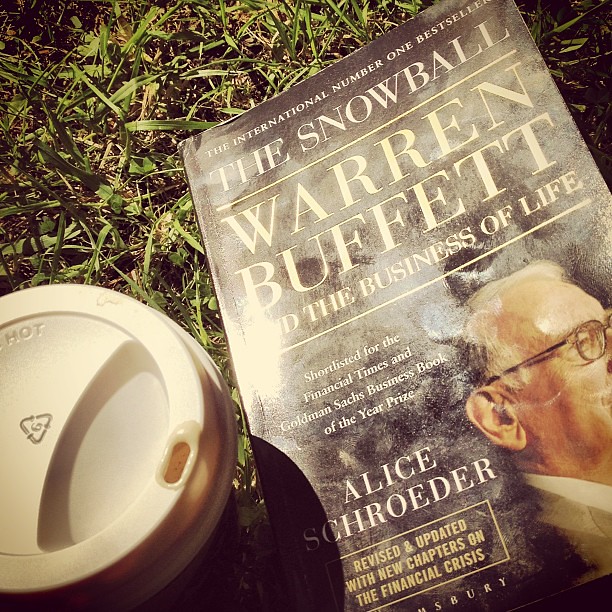In this detailed photograph, a book is prominently displayed on a green lawn, placed diagonally. The cover of the book is black and features a profile image of Warren Buffett, who is wearing glasses and a gray suit. The book's title, "The Snowball," is written in bold white letters with a yellow underline. Below the title, in smaller white letters, it reads, "Warren Buffett and the Business of Life." Near the bottom, the author's name, Alice Schroeder, is presented in white text. It further notes that the book is an "International Number One Bestseller" and was "Shortlisted for the Financial Times and Goldman Sachs Business Book of the Year Prize." Additionally, there is a yellow-outlined box stating that the book is "Revised and Updated with New Chapters on the Financial Crisis." Situated in the bottom left corner of the image is a white-lidded coffee cup, which appears to have a dark-colored body. Engraved on the lid are the words "hot" and a recycling symbol with the number six. The sunlight casts a subtle glow on the whole scene, adding warmth to the image.